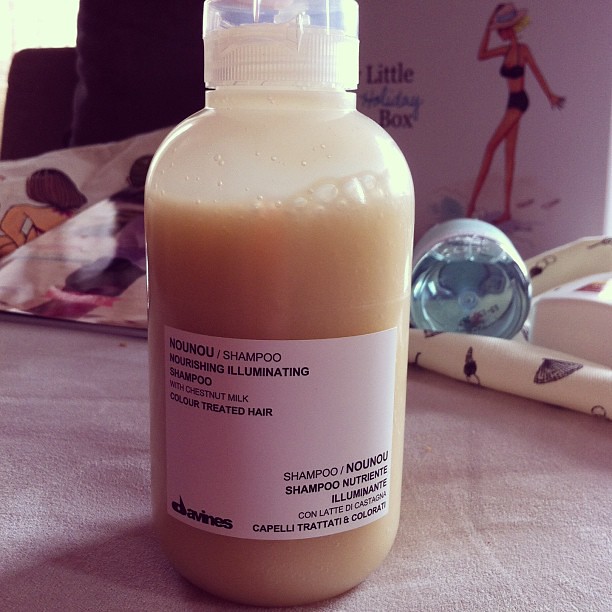The image showcases a close-up of a small, transparent bottle of shampoo containing a light tan or beige liquid. The plastic bottle, adorned with a plain white label featuring black text, prominently advertises "NOUNOU Shampoo" identified as a nourishing, illuminating shampoo with chestnut milk, specially designed for color-treated hair. Additionally, the lower section of the label displays the Italian translation: “Shampoo Nutrient Illuminante con Latte di Castagna.” The brand "Davines," spelled D-A-V-I-N-E-S, appears in green text in the lower-left corner of the label. The bottle is resting on a pink towel or tablecloth. Behind it, a package lies flat, displaying the label "Little Holiday Box" with a drawing of a woman in a bikini, her hand on a hat, standing on a beach. The setting also includes a rolled-up cloth with some text and a calendar or picture in the upper background depicting a woman in green shorts.